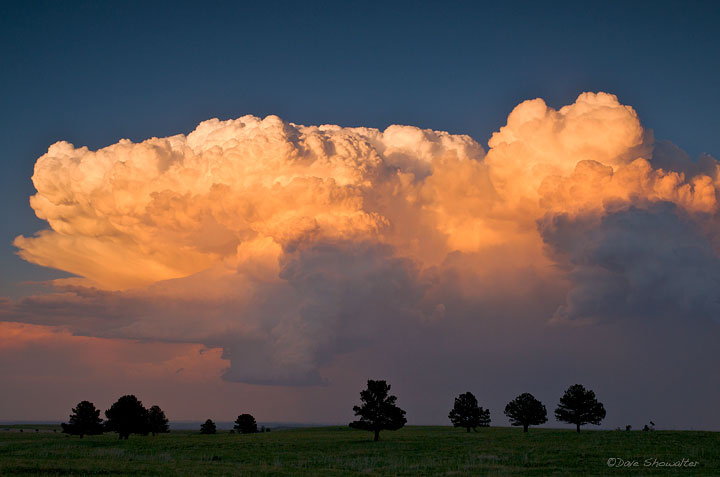This vibrant outdoor photograph, captured in landscape mode, showcases a striking, dramatic sky over a green field dotted with silhouetted trees. The very top third of the image features a deep, dark blue sky, while a massive cloud formation dominates the center. The clouds exhibit a stunning ombre effect, transitioning from bright white at the top to a vivid orange lower down, due to the sun's light casting an ethereal glow. Below the orange hue, the clouds darken to almost black, suggesting the onset of a storm, with the potential for rain hinted by the blurred appearance near the bottom. Framing the bottom of the image is a lush field of grass, interspersed with unevenly spaced trees—four on the right, five on the left, amounting to nine trees in total. In the lower right-hand corner, the photograph is subtly signed in cursive with the name "Dove Shoa Walter," crediting the artist. This image masterfully blends elements of serene beauty and impending natural power.